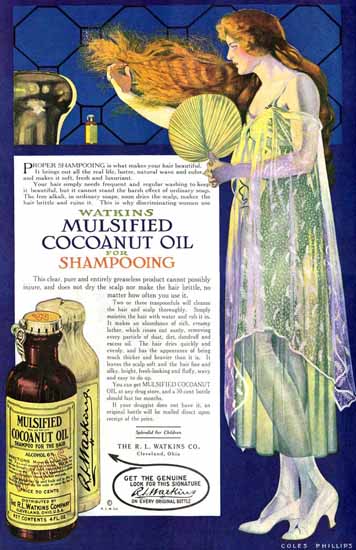The image is a vintage advertisement for Watkins Emulsified Coconut Oil Shampoo. The backdrop is a dark blue, featuring a chain link fence pattern and black shapes resembling pinecones or honeycombs. A distinguished woman with long, wavy hair—varying descriptions suggest she could be blonde or red-haired—adorns a sheer, flowing gown and white high heels. She gracefully holds a fan in her hands. Alongside her, prominently displayed are two old-fashioned bottles of the shampoo, featuring brown and white containers with pop lids. The ad headline reads "Watkins Emulsified Coconut Oil for Shampooing," with the word "coconut" intriguingly spelled "C-O-C-O-A-N-U-T." Additional text mentions achieving a genuine look but is difficult to read due to photo resolution. The aesthetic and details hint that the advertisement is from the early 1900s, encapsulating a nostalgic charm.